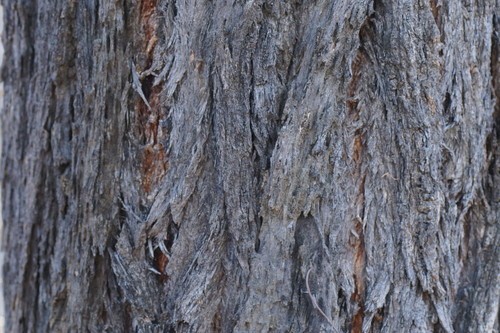This image is an extreme close-up of a tree trunk, revealing intricate details of its bark. The bark appears to be shedding, either due to the tree's natural life cycle or its specific species characteristics, such as hickory, ironbark, or acacia. The texture of the bark is dry and rough, displayed in a grayish hue with underlying tones of brown. Some sections of the bark have begun to peel and break off, especially noticeable towards the left side where the revealed area appears orange, and to the right side where it has a reddish tint. These peeling sections give the impression of being shaved off, accentuating the rugged texture. There is a distinctive small V-shaped mark in the middle of the trunk. The close-up nature of the photograph obscures any background or context, emphasizing the vertical direction of the bark and the sizable girth of the tree. The image includes no signs of insects, birds, or other external elements, focusing solely on the tree's bark.